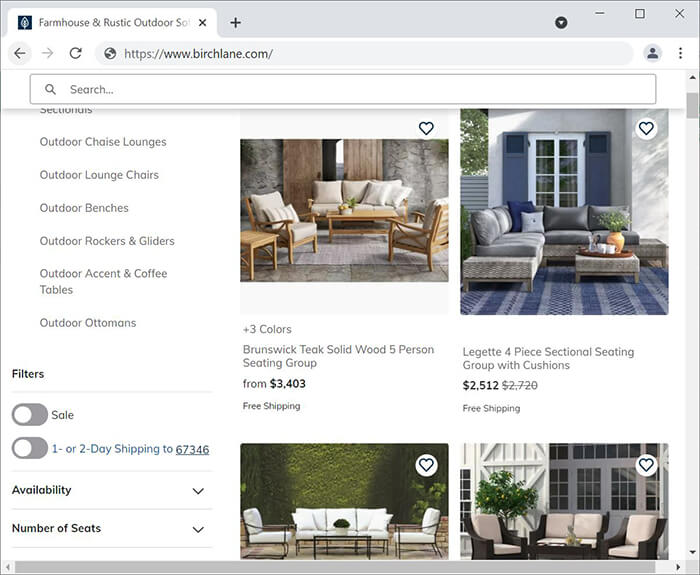Screenshot of a desktop browser window open to the Birchlane.com website, featuring a tab titled "Farmhouse and Rustic Outdoor." At the top of the webpage, there's a static search bar that remains visible as you scroll. On the left side of the screen, a navigation menu offers various outdoor furniture options such as outdoor chaise lounges, outdoor lounge chairs, outdoor benches, outdoor rockers and gliders, outdoor accent and coffee tables, and outdoor ottomans. Below these categories, there are filter options for sale items or one- to two-day shipping, as well as filters for availability and the number of seats. On the right side of the page, images and listings of products are displayed, including items like the "Brunswick Teak Solid Wood Five-Person Seating Group" priced at $3403.